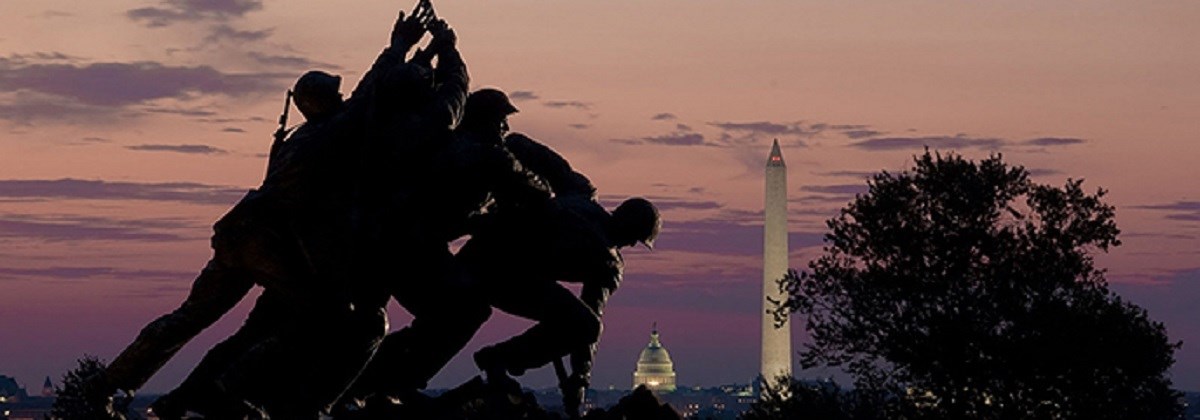This stunning panoramic photograph, taken in Washington, D.C. at dusk, captures the iconic Iwo Jima Memorial in dramatic silhouette against a vibrant sunset sky. The breathtaking gradient of colors transitions from light purples and pinks at the top, deepening to darker purples and blues towards the horizon. The silhouette of the six soldiers raising the American flag at Iwo Jima is sharply outlined, highlighting the high-quality, artistic nature of the shot. In the background, the majestic Washington Monument, with its unmistakable obelisk shape, and the large dome of the Capitol Building are clearly visible, affirming the location. A large tree stands next to the Washington Monument on the right, adding an element of natural beauty to the scene. This richly detailed image not only emphasizes the memorial but also beautifully captures the essence of Washington, D.C.'s historic skyline, making it a perfect candidate for a tourist brochure.